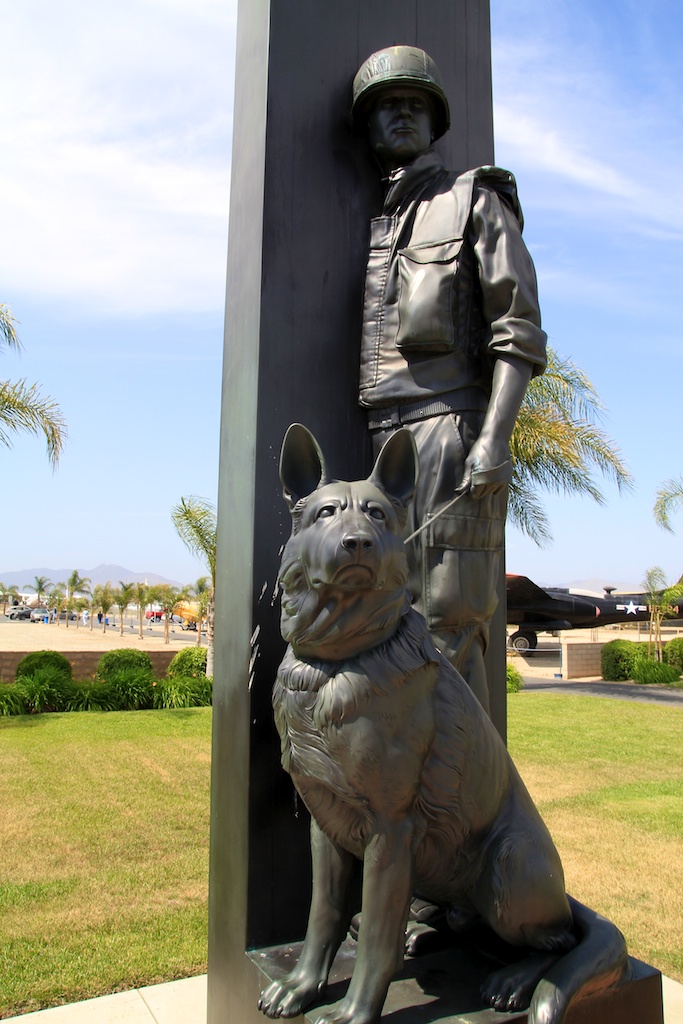This photograph captures a striking outdoor sculpture, prominently centered in the image, set against a backdrop of lush green grass and a scenic beach area adorned with palm trees under a clear blue sky. The dark-colored, possibly black, monument features a soldier, garbed in a detailed army uniform complete with a tactical vest and helmet. The soldier, emerging from a gray wall, holds the leash of a German Shepherd, which stands or sits alertly at his feet, its ears perked up and eyes fixed on the distance. The finer details of the soldier, such as his rolled-up long-sleeve shirt and multiple-pocket jacket and pants, add to the lifelike quality of the sculpture. The sculpture is elevated on a podium, enhancing its stature within the park. Although the man's face is shadowed, the overall composition emphasizes his protective stance beside the attentive dog. In the background, the blurring of shrub bushes and a distant road maintain the focus on the powerful, solemn memorial, likely commemorating the bond and bravery of soldiers and their canine companions.